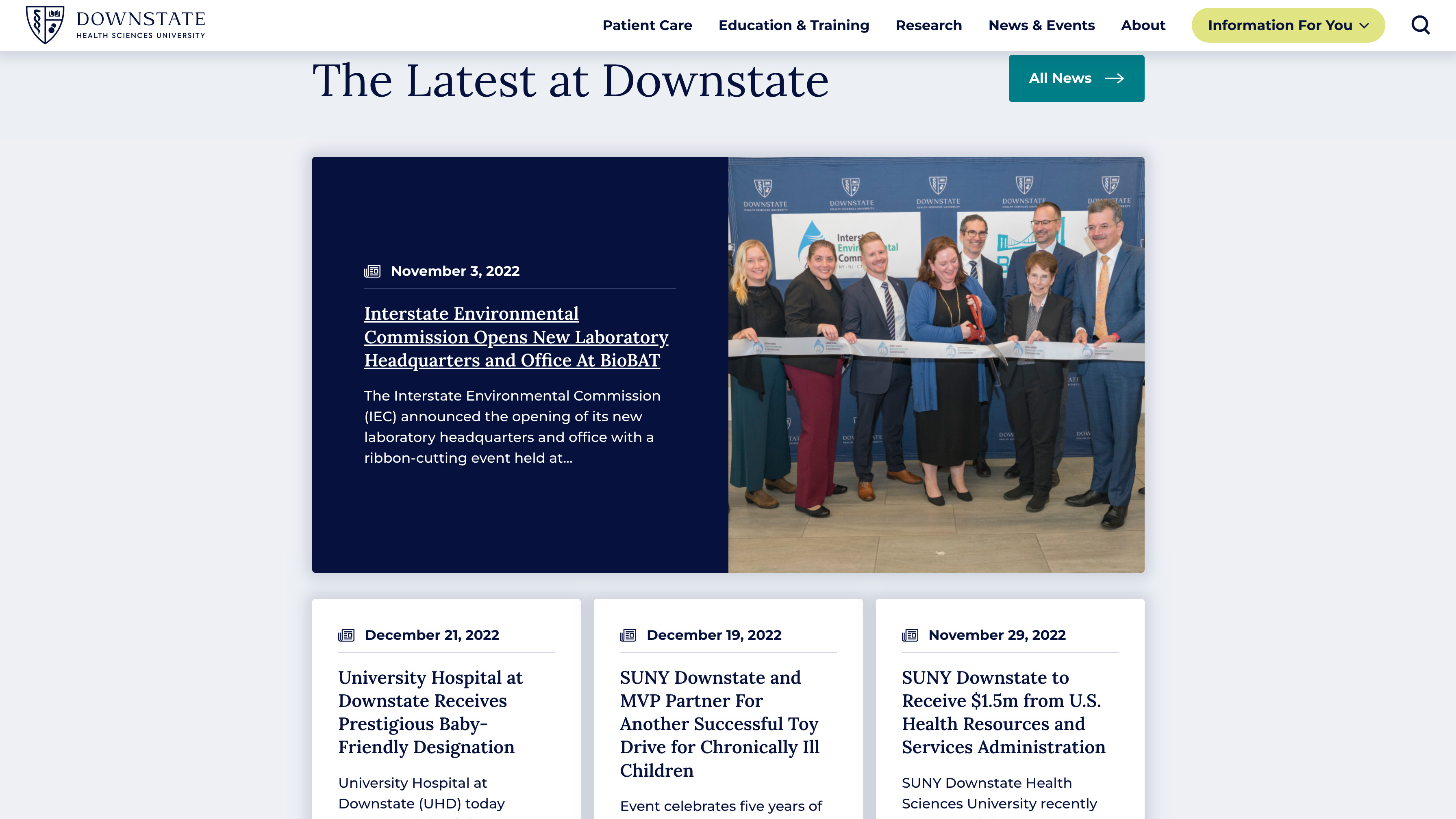In an image captured during the ribbon-cutting event, a group of people, led by a prominent figure holding a pair of scissors, celebrates the grand opening of the Interstate Environmental Commission's new laboratory headquarters and office at BioBat. The event, held on November 3rd, 2022, marks a significant milestone for the Commission. A large ribbon spans the front of the group, emphasizing the ceremonial occasion. The photograph also reveals a headline confirming the Commission's announcement, while below it, three additional articles are highlighted. These articles detail the University Hospital at Downstate receiving a prestigious baby-friendly designation, an account of a successful toy drive, and news of a $1.5 million grant awarded by the U.S. Health Resources and Services Administration.